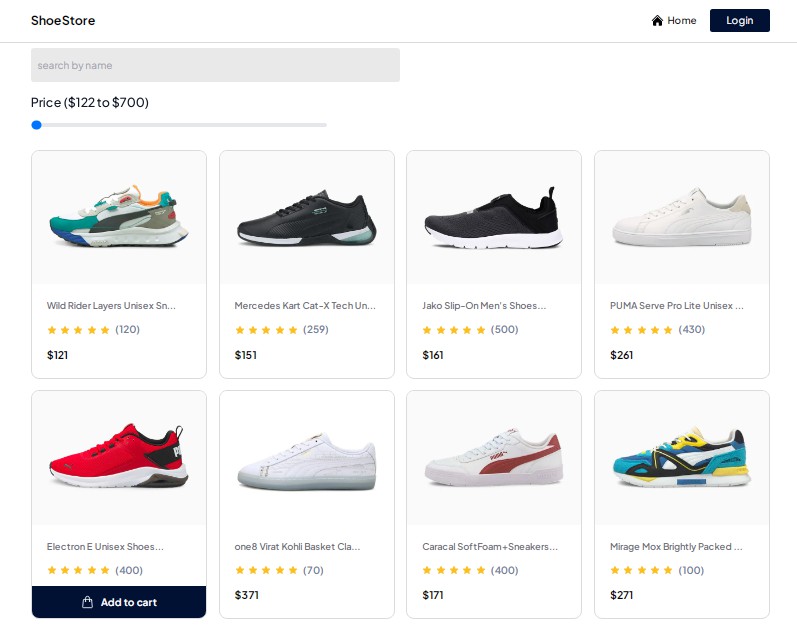The image is a screenshot taken from an online web page of a shoe store. The webpage features a clean, white background and prominently displays eight different images of sneakers arranged in two rows with four sneakers each. 

In the upper left corner of the webpage, the words "Shoe Store" are written in black. Just below this, there is a gray search bar with the placeholder text "Search by name". Directly below the search bar, the price range is indicated, stating "$122 to $700".

In the first row, starting from the left:
1. A multicolored sneaker featuring shades of green, white, black, red, and yellow.
2. A white and black sneaker.
3. Another white and black sneaker.
4. A pure white sneaker, with the price of $261 displayed beneath it.

In the second row:
1. The first sneaker is red and white in color.